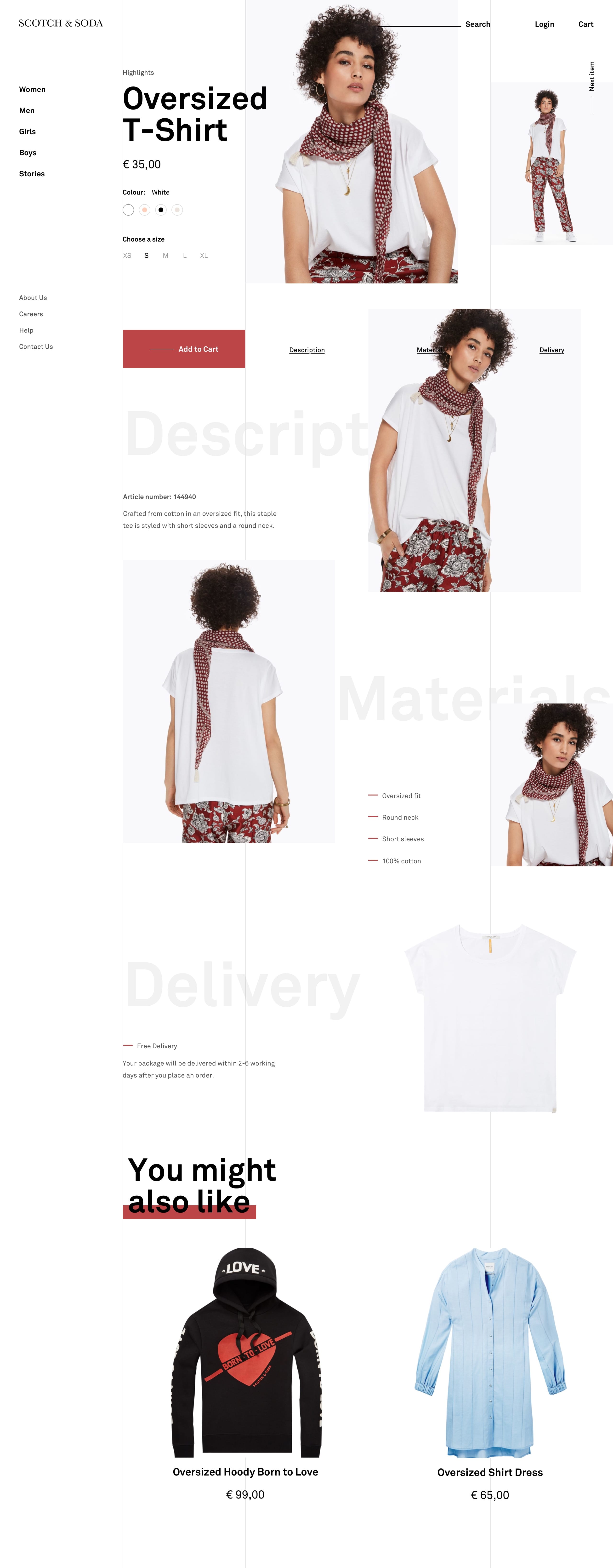This e-commerce webpage showcases a women's oversized white t-shirt, modeled by a woman with darker skin and curly hair. She is featured in five different photographs, highlighting various aspects of the t-shirt. The model pairs the t-shirt with a knit scarf and floral print pants, demonstrating a stylish and versatile look. At the top of the page, the product name "Oversized T-Shirt" is prominently displayed, along with its price beneath it. A red button, likely a 'Buy' button, invites customers to make a purchase. Lighter, semi-transparent text serves as the background, with headlines such as "Description," "Materials," and "Delivery," each accompanied by small, unreadable bulleted text. At the bottom of the page, there is a section titled "You Might Also Like," showcasing two additional items, either sweatshirts or a robe. The experienced model effectively poses, enhancing the appeal of the t-shirt for potential buyers.